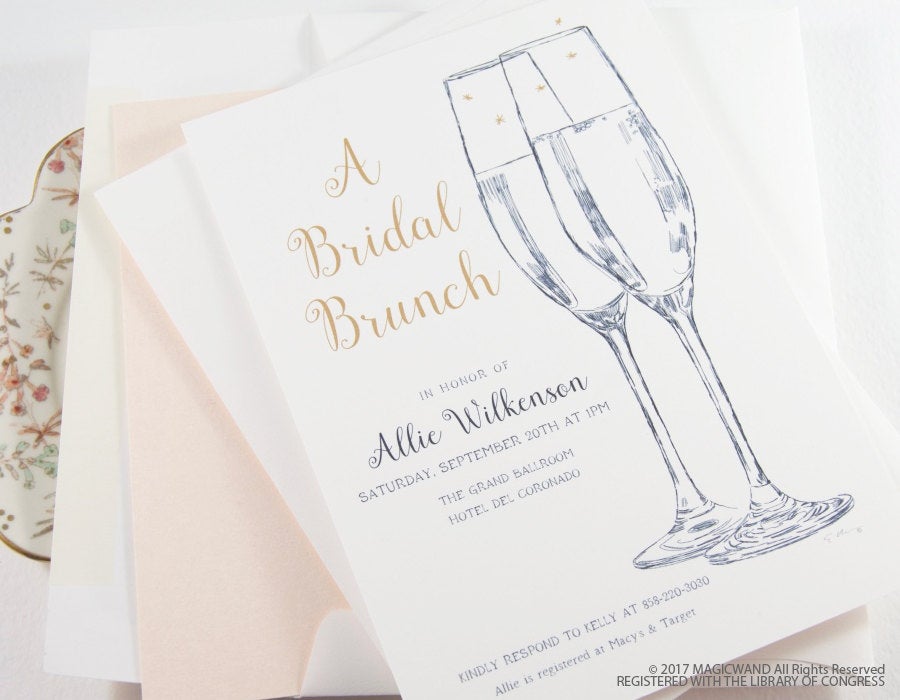This is an elegant invitation to a bridal brunch in honor of Allie Wilkinson. The event is scheduled for Saturday, September 20th at 1 p.m. and will take place in the Grand Ballroom of the Hotel Del Coronado. The invitation, which features both light brown and black writing, prominently displays two champagne glasses adorned with subtle gold design accents. It asks guests to kindly respond to Kelly at 858-220-3030 and notes that Allie is registered at Macy's and Target. The background of the invitation has a soft pink hue. At the bottom, a trademark states "2017 Magic Wand, All Rights Reserved, registered with the Library of Congress." The invitation is placed on a table, accompanied by a peach-colored envelope and additional papers, all resting on a gold-embroidered, white ceramic plate with a floral design around the edge. The overall presentation exudes sophistication, with the champagne flutes and the soft linen-like napkins adding to its refined appearance.